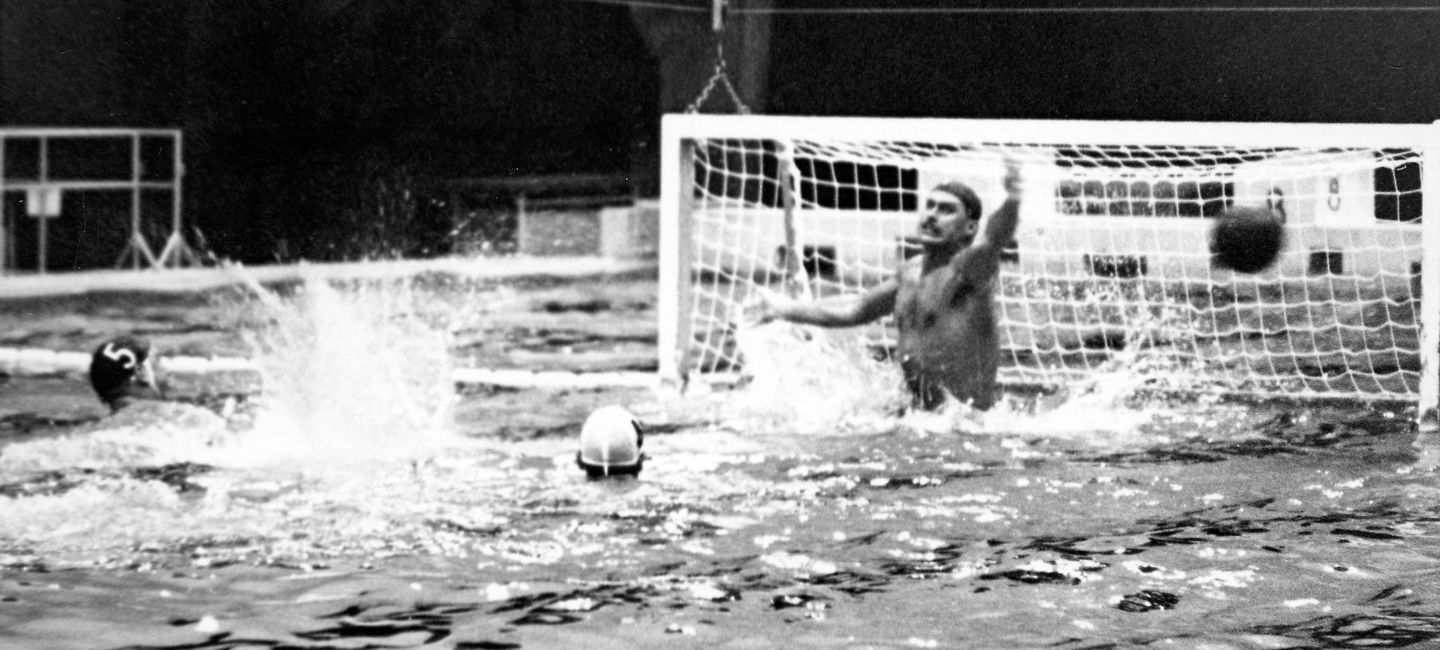This black-and-white photograph captures a historic moment in a water polo match, likely from an earlier era given its grainy texture. The scene is set in a swimming pool, centered around a goalpost that dominates the right half of the image. The goal, with its white frame and matching net, seems roughly the height of a person's upper body and extends backward in a rectangular shape. 

A muscular goalie, with a close-cropped hairstyle or a swim cap and a distinct mustache, is seen leaping out of the water in a dramatic attempt to block the water polo ball, which is captured mid-air to his right and appears to be heading into the net. His arms are fully stretched out, showcasing his athletic build. 

To the left of the goalie, partially submerged in the water, are two other players. The one closest to the goalie wears a white swim cap and is primarily visible from the neck up, looking away from the camera, making their features hard to distinguish. Further left is another player, visible from the shoulders up, who wears a dark swim cap marked with the number 5.

The backdrop features a pool deck and a dark wall, with a metal railing partially visible in the upper left corner. Additionally, a few crates or plastic containers are scattered along the pool's edge, adding to the vintage ambiance of the scene.